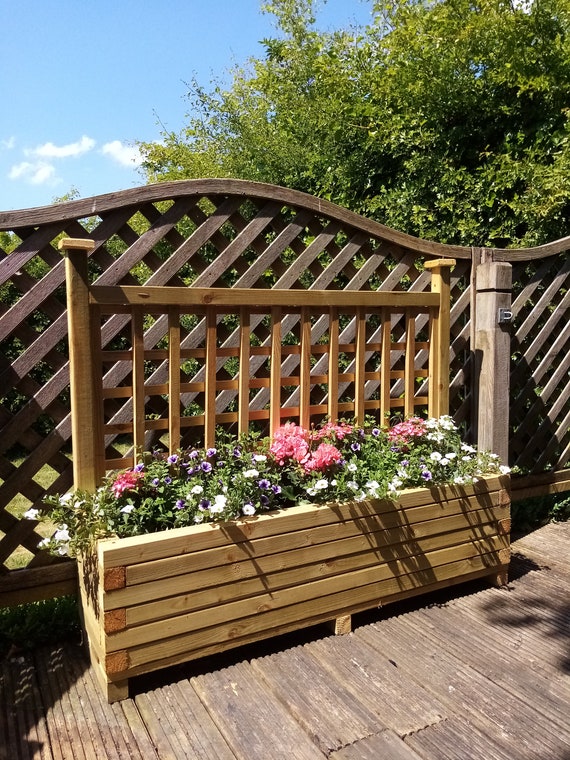The image depicts an outdoor scene, likely someone's backyard, centered around a detailed wooden flower bed or planter. The wooden structure features seven horizontal slats, arranged in a distinctive pattern where the second, fourth, and sixth bars show their square ends from the sides. The planter has a high frame with a slight metal lining, and various colorful flowers spilling out from it. The flowers are arranged in a gradient, with white flowers on the left, followed by mixed red and purple flowers towards the center, and red and white flowers on the right. Surrounding the flower bed is a wooden fence or deck, adding to the rustic charm with its darker brown tones. The backdrop includes tall, open-spread trees and a vibrant blue sky with clouds, complementing the scene with lush green scenery. The major colors in the image include various shades of green, brown, white, blue, peach, pink, red, and purple, all contributing to a vivid and detailed garden tableau.